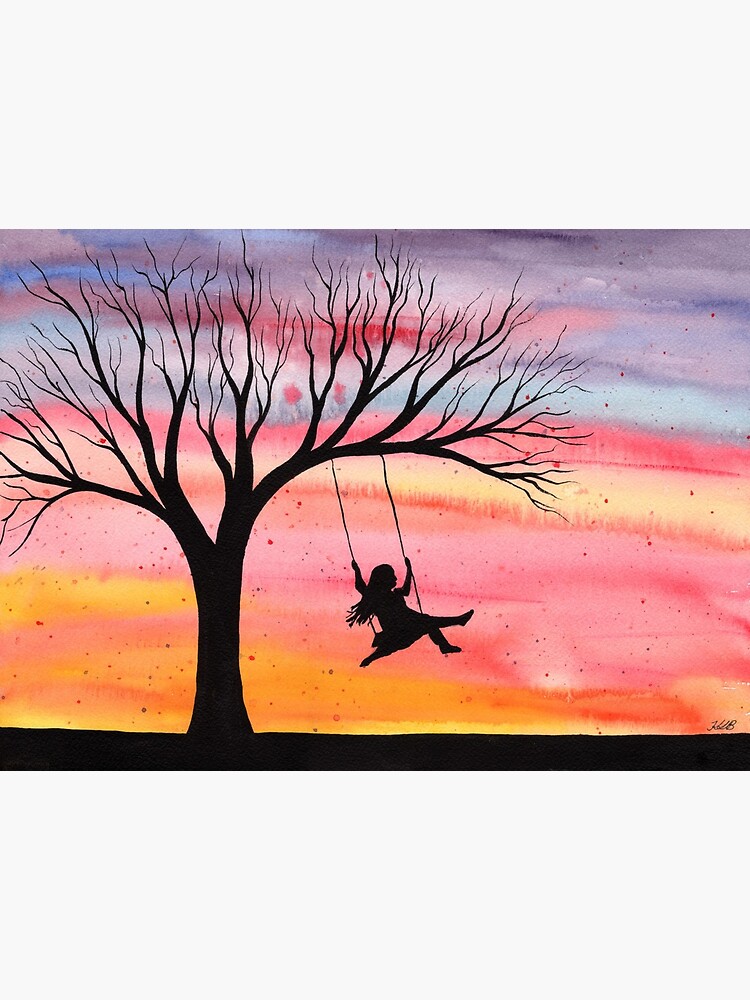In this evocative image, a young girl swings from a tree, both captured in silhouette against a breathtaking sunset. The tree, devoid of leaves, and the swing create striking black contrasts against the vibrant, watercolor-like sky. The sunset hues—red, orange, yellow, blue, and purple—blend seamlessly, interspersed with splatters of the same vivid colors, lending a dynamic, painterly feel to the scene. The girl's hair blows in the wind, one foot extended joyfully while the other dangles, capturing a carefree moment steeped in beauty and simple pleasures. The ground beneath is also silhouetted, grounding the ethereal composition. Rendered with a semi-cartoon style, this piece exudes charm and whimsy, marked with the artist's signature in the bottom right corner.